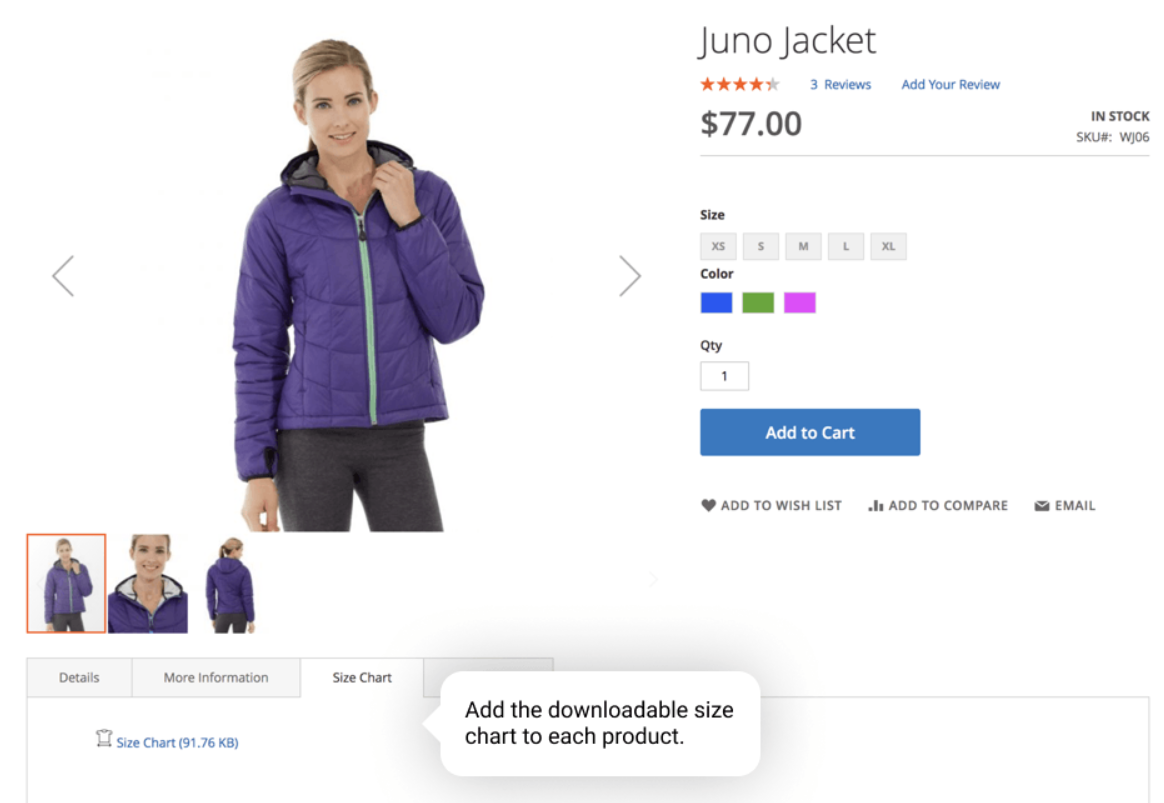The image showcases a product page from a website with a clean, white background. On the left and right sides of the center, there are arrows pointing left and right, respectively. Positioned between these arrows is a full-body image of a woman modeling a jacket. 

The woman is dressed in black leggings and a purple puffer jacket with a hood. The interior of the jacket is black, and it features a mint green zipper that extends up to the collar. The woman has her left hand raised towards her collar as if adjusting the jacket.

Beneath the main image, there are three smaller images displaying different views of the jacket. Below these images, the website provides several options: "Details," "More Information," and "Size Chart." The size chart is shown, along with a prompt to download the size chart for each product.

On the right side of the page, product details are listed. The item is called the "Juno Jacket," with both words capitalized. There is a star rating graphic accompanied by text indicating "Three Reviews" and a link to "Add Your Review." The jacket is priced at $77, and the available sizes are Extra Small, Small, Medium, Large, and Extra Large. The available colors are described as blue-purple, green, and purpley magenta.

Below this, there are options for selecting the quantity (QTY 1), and buttons for "Add to Cart," "Add to Wishlist," "Add to Compare," and "Email."